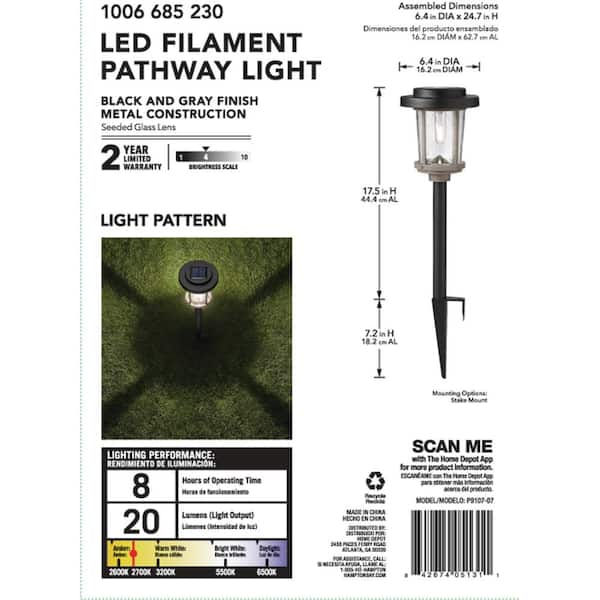**Descriptive Caption:**

This is an image showcasing a LED filament pathway light, a type of outdoor lighting designed to illuminate pathways and gardens at night. The light features a mini lantern design with a stake at the bottom, allowing it to be easily inserted into the ground for stability. Constructed from metal with a black and gray finish, the light includes a seated glass lens for added durability and aesthetic appeal.

Highlighted in the image is a sticker with detailed product information. The light boasts a 2-year limited warranty, operates for up to 8 hours, and has a light output of 20 lumens. Dimensionally, it measures 6.4 inches in diameter and stands 24.7 inches tall. In one corner of the image, there's a barcode with the instruction "scan me," indicating that additional product details can be accessed via the Home Depot app. The image also includes a visual of the pathway light in use, firmly placed in the ground and surrounded by grass, demonstrating its practicality and ambiance-enhancing qualities.